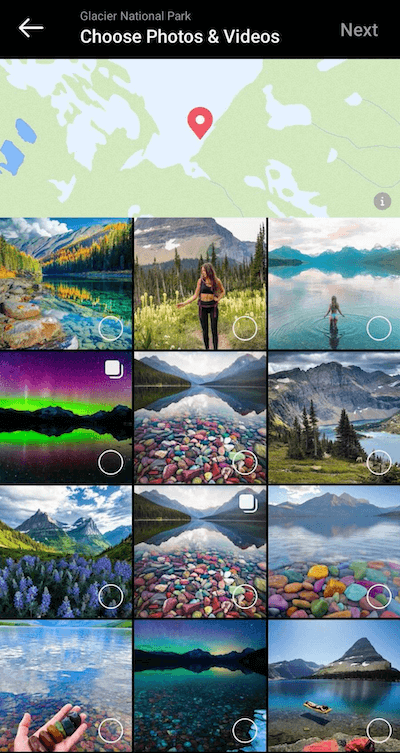The image displays various options for pictures within a mobile interface. At the top, a black horizontal bar features a white arrow pointing to the left, and in the center, smaller white text reads "Glacier National Park." Bold white text below it instructs users to "Choose photos and videos," while the top right corner contains the word "Next" in light gray.

Below this top bar, a faint map is visible, predominantly in light yellow and white, presumably representing land areas. A light red location symbol is positioned centrally on the map. On the bottom right of the map, a gray circle with a white eye icon in the center indicates a viewing option.

At the very bottom of the image, there is a 3x4 grid displaying a selection of photos. Each photo features a small circle in the bottom right corner. Notably, the first picture in the second row and the middle picture in the third row both have an emblem resembling a stack of two overlapping squares in their bottom right corners.